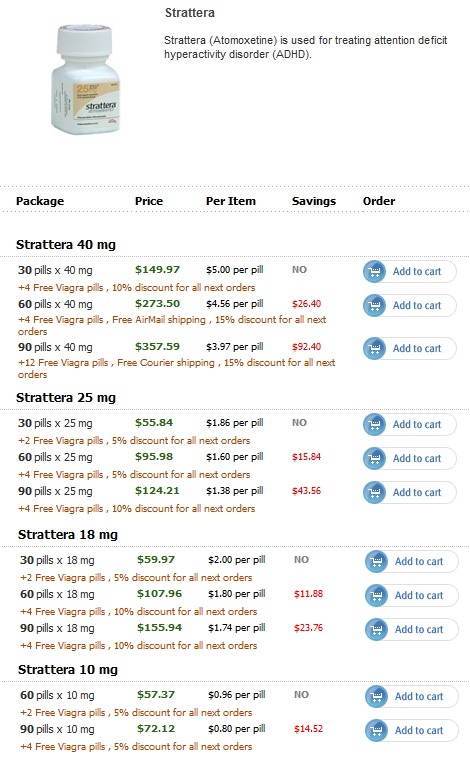The image is a web screenshot displaying information about a drug called Strattera. In the upper left-hand corner, there is a photograph of a Strattera bottle, characterized by its somewhat square base and a twist-off cap. To the right of the image, the name "Strattera" is prominently displayed, spelled out as S-T-R-A-T-T-E-R-A.

Below the drug name, a brief description states that "Strattera" is used for treating attention deficit hyperactivity disorder (ADHD). Following the description is a tabulated list, which includes columns for the package type, price per item, savings opportunities, and order options.

Further down the page, there are sections dedicated to various dosage options available for Strattera, including 40mg, 25mg, 18mg, and 10mg options. Each dosage option likely has additional details on pricing and ordering specifics, although these details are not explicitly described in this caption.